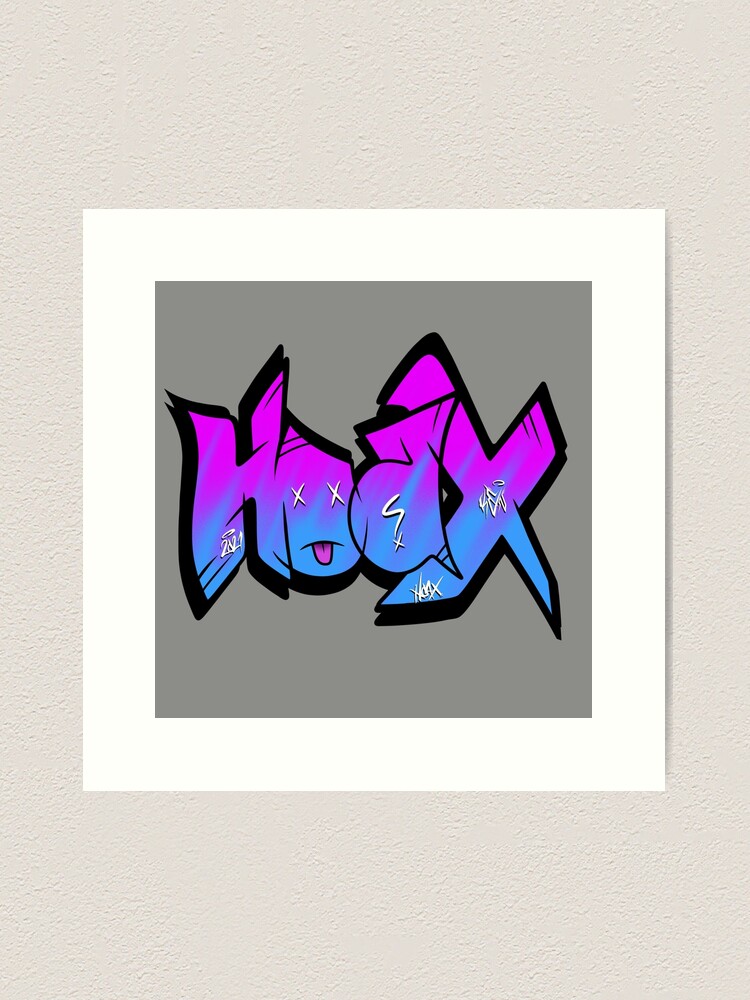The image depicts a vertically aligned rectangular artwork hanging on an ivory-textured wall, framed by a thick, flat, white frame. The centerpiece of this artwork is a solid dark gray square background that contains large, graffiti-style bubble letters spelling out "HOAX." The top half of the letters is painted in purple, while the bottom half transitions into a blue hue. The letters are outlined in thick black lines, giving them a bold appearance. Notably, the letter "O" is illustrated with a face, featuring two white X's for eyes and a pink tongue sticking out, imitating a playful, cartoonish look. Additionally, the letter "A" incorporates a design resembling a question mark with an X replacing the dot below it. The entire composition is dynamic and evokes a street-art aesthetic, highlighted by subtle white symbols and signatures possibly from the artist on the "H" and the "X."